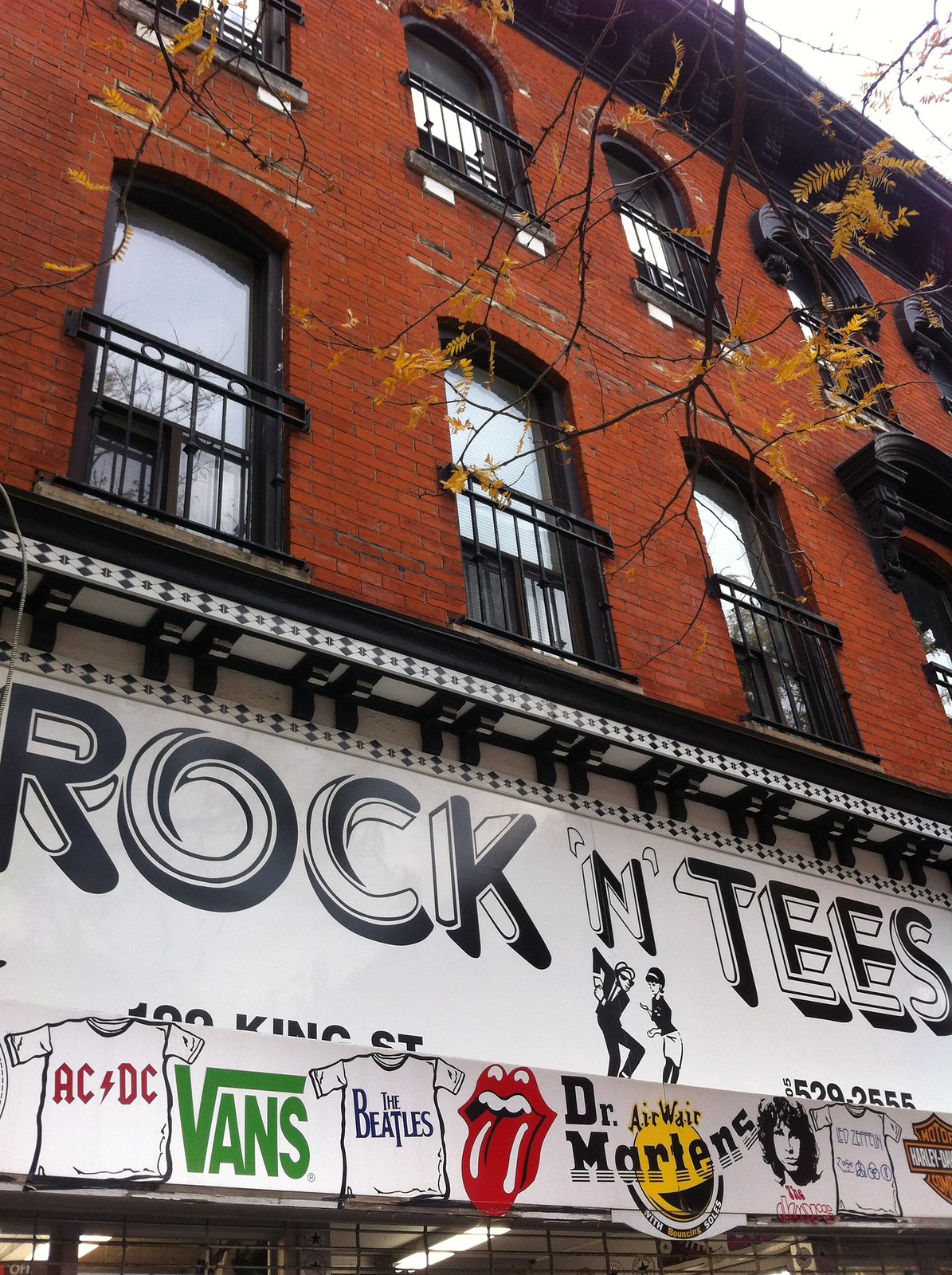The image showcases the front of a large, vintage-style building that appears to be at least three stories high. The top two stories feature a brick façade adorned with vertical, arched windows that resemble Juliette balconies equipped with railings. The roof is dark blue and is partially adorned with trees and bushes, some with yellow leaves. 

On the first floor, the building prominently displays a white marquee with the text "Rockin' Tees" in black font. Below this sign, there are various logos and images of t-shirts. From left to right, the signage includes an ACDC t-shirt, the Vans logo in green, a The Beatles t-shirt, the iconic Rolling Stones lips, the Doc Martens logo, The Doors t-shirt, and the Harley Davidson emblem. Additionally, there is a white billboard above the marquee with partial images of a man and a woman dancing in the center, and partial text indicating the location details, such as "Hundred King Street" and a phone number ending in "5293355."

The lower part of the building appears to be the entrance to a shop or showroom, equipped with big lights in the ceiling, enhancing the commercial focus of this part of the building.